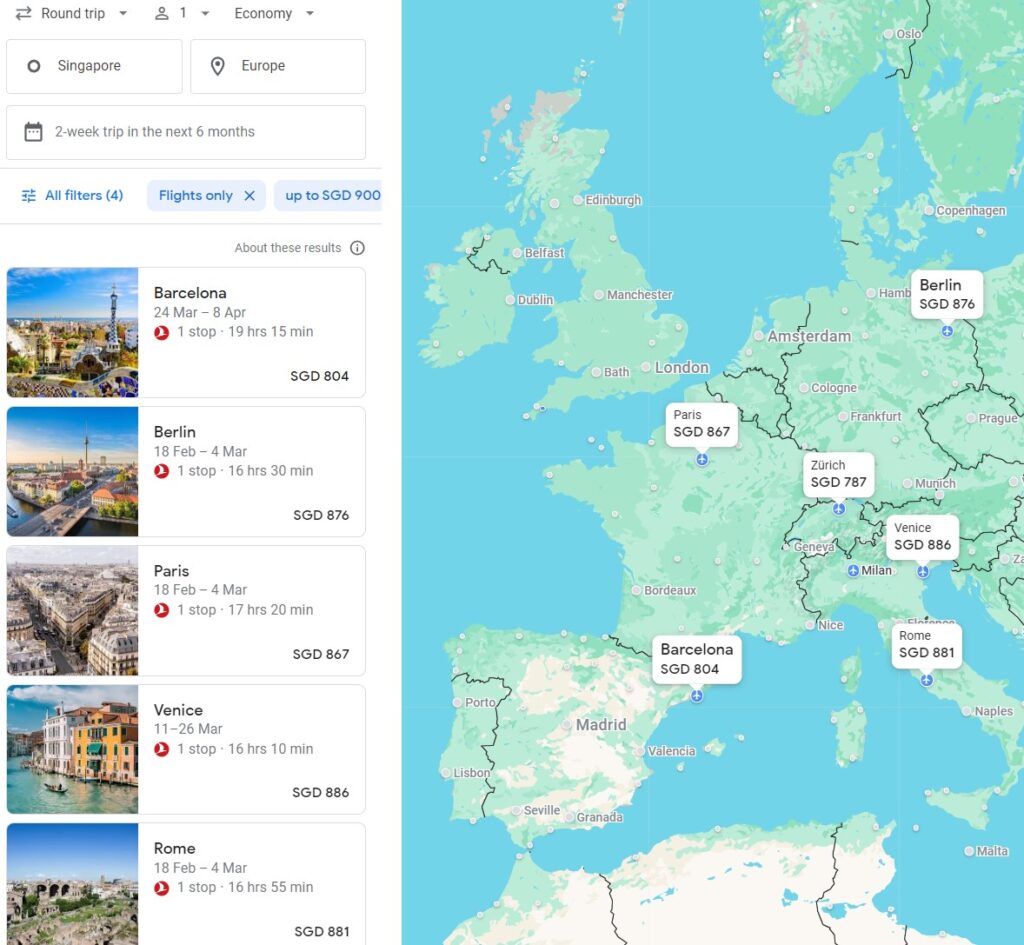This detailed Google Maps image of Europe occupies about 60% of the right page of a split-screen view. The left page features a detailed trip planner interface with various travel information.

At the top of the left page, there are travel options marked with small icons: a round-trip option, a person icon indicating economy class, and buttons for Singapore and Europe, the latter with a pin icon. Beneath this, there is an option to take a two-week trip in the next six months, marked by a calendar icon. Below this, the 'All Filters' button is highlighted in blue, followed by tags for 'flights only' and a budget cap of 'up to SGD 900'.

Highlighted cities on the map include Barcelona, Berlin, Paris, Venice, and Rome, each represented with a corresponding number and specific information:
- **Barcelona**: SGD 804, from 24 March to 8 April, one-stop flight lasting 19 hours and 15 minutes.
- **Berlin**: SGD 876, from 18 February to 4 March, one-stop flight lasting 16 hours and 30 minutes.
- **Paris**: SGD 867, from 18 February to 4 March, one-stop flight lasting 17 hours and 20 minutes.
- **Venice**: SGD 886, from 11 March to 26 March, one-stop flight lasting 16 hours and 10 minutes.
- **Rome**: SGD 881, from 18 February to 4 March, one-stop flight lasting 16 hours and 15 minutes.

Zurich is also marked on the map, although it is not listed on the left side with the other cities. 

The map itself prominently features Rome in the center, with European countries separated by black lines, cities marked with dotted points, and bodies of water rendered in blue. The map extends to show parts of North Africa as well.